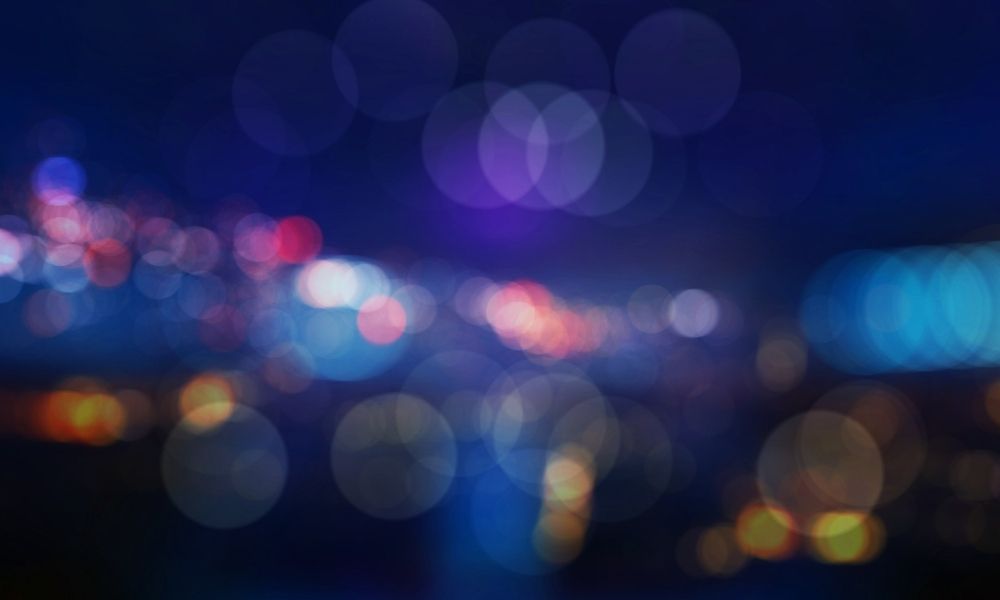The image is a highly blurred nighttime photograph, reminiscent of how scenes appear when one squints or has astigmatism. It features a series of overlapping, translucent colored circles against a dark background, possibly black or dark blue, evoking the appearance of headlights or taillights. Predominantly in the center are circles in shades of pink, red, purple, and blue, varying in size. On the right side, larger blue concentric circles are evident, while smaller yellow circles form a line at the bottom. Above these are more translucent white circles scattered across the top and bottom. The overall effect is a dynamic, abstract blend of intersecting colors and shapes that create a kaleidoscopic night scene.